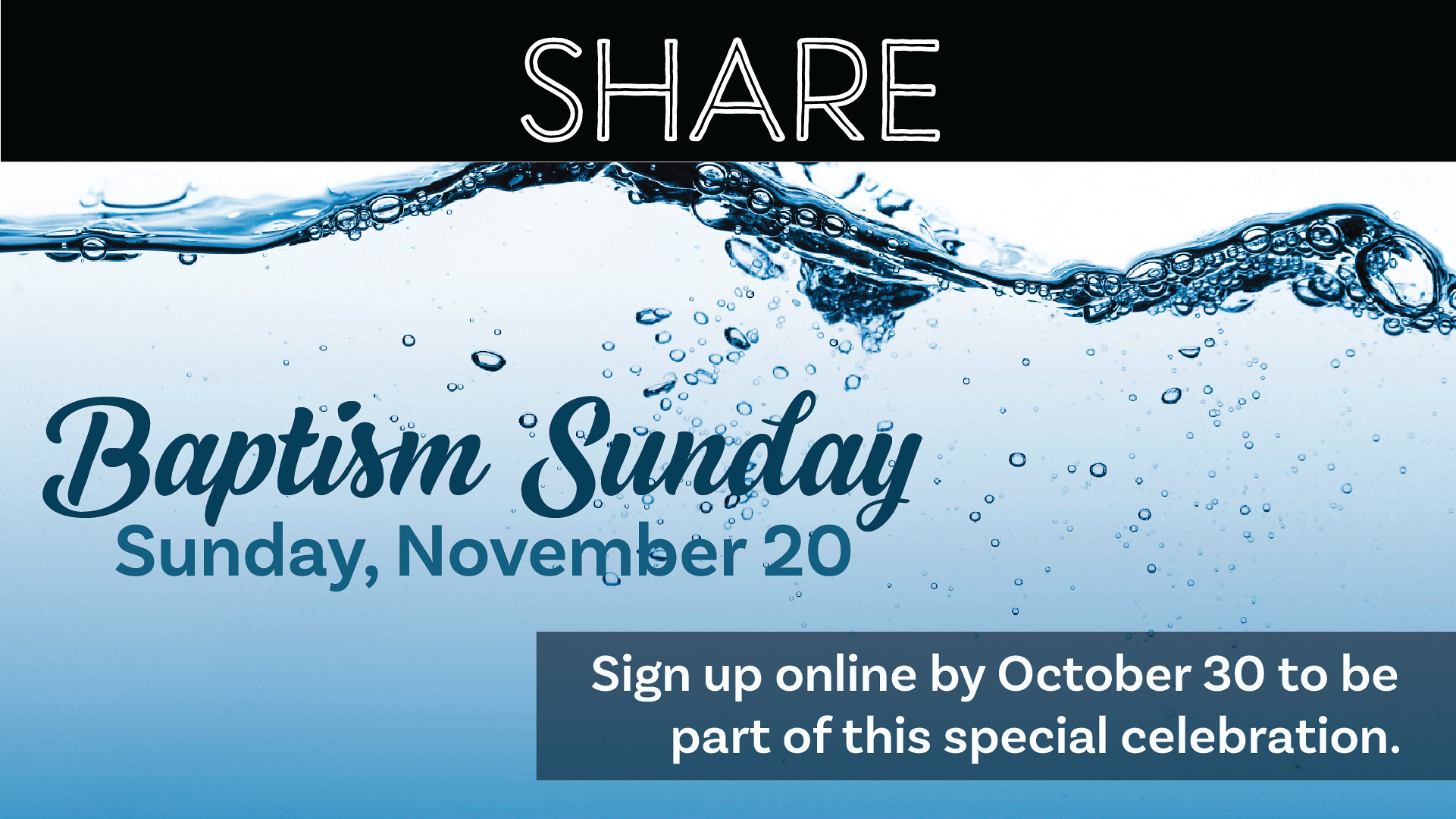The image is a rectangular landscape with a prominent black header at the top featuring the word "SHARE" in bold, all-cap white letters with thin black strips inside each letter. Below the header, the scene transitions into a clear blue underwater view. The waterline at the top is depicted with realistic waves and bubbles, emphasizing the aquatic theme. In the center-left, the words "Baptism Sunday" are written in elegant, dark blue cursive. Directly beneath this, in a slightly lighter blue print, the date "Sunday, November 20th" is displayed. Towards the lower right, a dark blue rectangular box contains white text that reads, "Sign up online by October 30th to be part of this special celebration." The overall design conveys a serene and celebratory mood, fitting for an event like a baptism.